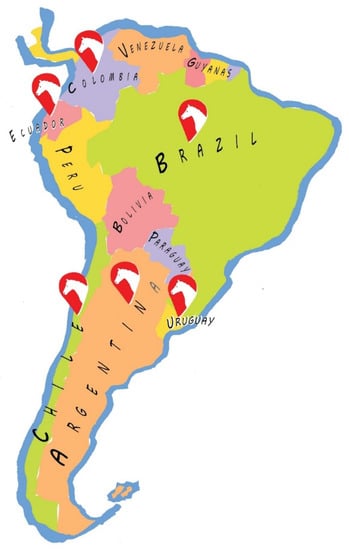This detailed and colorful map of South America highlights the continent's countries with each region distinctly shaded in various hues: Ecuador in pink, Colombia in purple, Venezuela in orange, Guyana in pink and orange, Brazil in light green, Peru in light yellow, Bolivia in pink, Paraguay in gray, Uruguay in yellow, Argentina in orange, and Chile in light green. The map is framed by a light blue border and set against a white background. Notably, it features five red teardrop-shaped graphics with white horse silhouettes, marking locations in Ecuador, Colombia, Brazil, Chile, and Argentina. The coloring scheme uses primarily green, orange, pink, and purple shades, with muted hues throughout. An island appears near the tip of the continent, though it remains unnamed. The map contains no additional text.